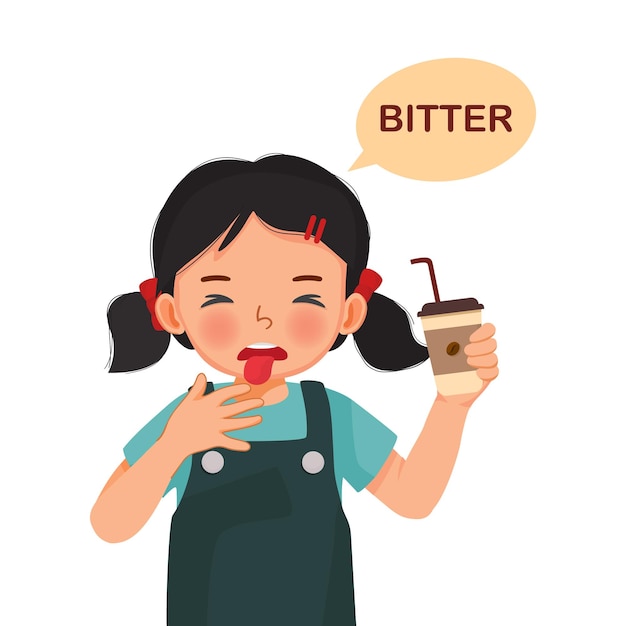The image portrays a cartoon drawing of a young girl with light tan skin and black hair styled in pigtails, adorned with red barrettes and ribbons. She has her eyes closed and her face expresses disgust, with two red blush circles underneath her eyes and her tongue sticking out. The girl is wearing a dark blue jumper with white buttons over a teal t-shirt. In her left hand, she holds a brown café-style cup with a brown wrapping for heat protection, a brown lid, and a brown straw. Her right hand is raised to her tongue attempting to wipe off the taste. Above her head, there is a peach-colored thought bubble with the word "bitter" written in brown lettering, capturing her reaction to the drink. The background of the image is white, focusing all attention on her expressive demeanor and adorable outfit.